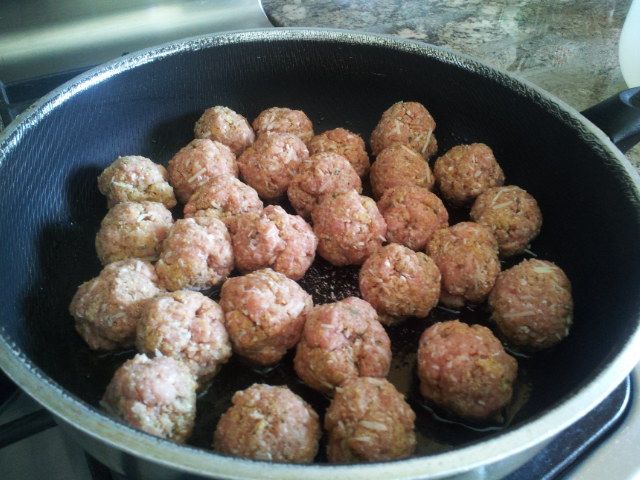This image captures a detailed view of a black, somewhat worn pan with a silver rim, situated on what appears to be a kitchen stove. The pan features a black handle extending from the upper right corner. Inside, arranged neatly in two circular patterns, are approximately 20 to 25 uncooked meatballs. The meatballs, potentially made of pork or beef and including grated cheese, are just starting to brown on one side, indicating that cooking has just begun. The interior surface of the pan is dark and has a serrated texture. The background of the image includes a glimpse of a stone-colored countertop and the lower portion of a black stove.